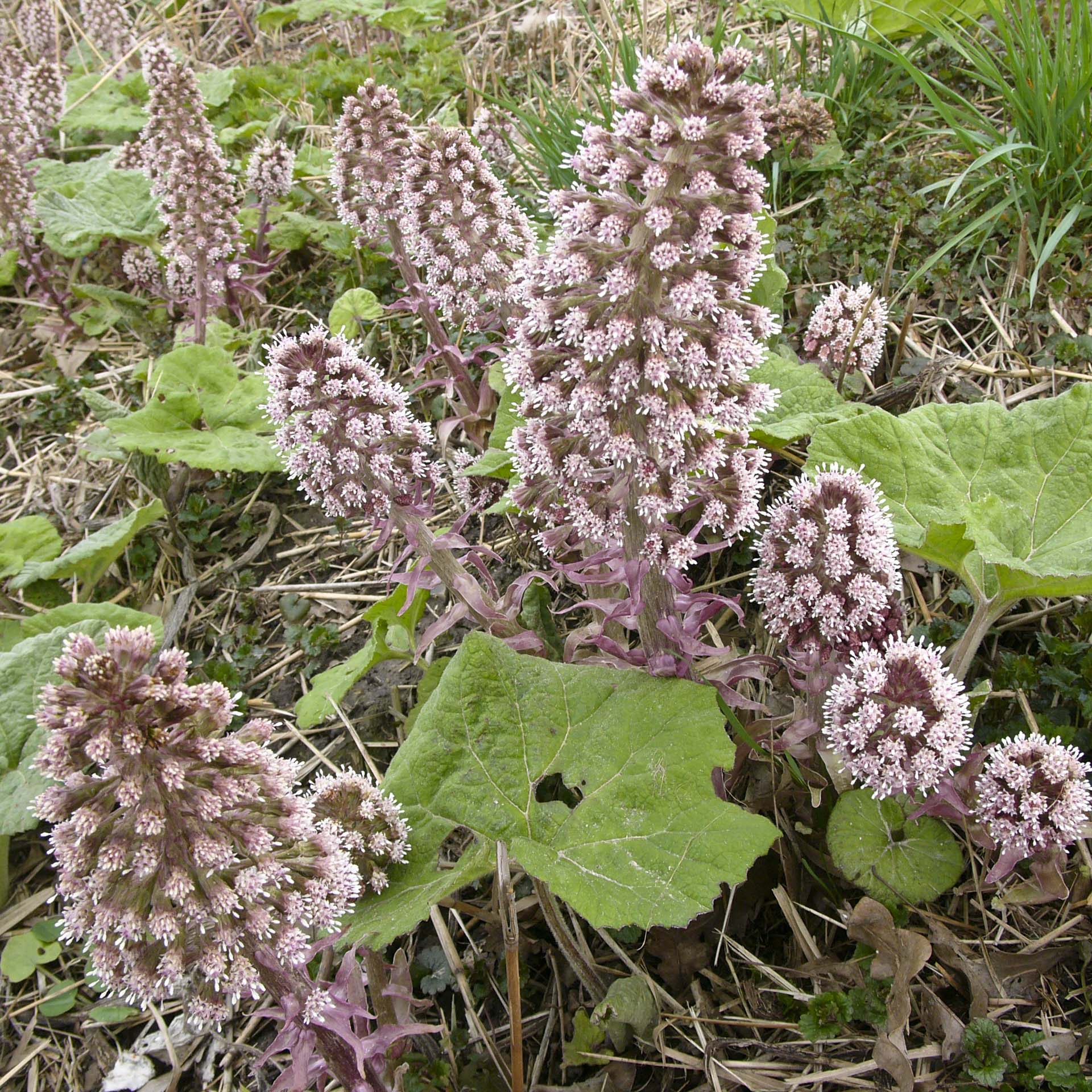The image showcases a close-up view of various plants amidst a wilderness setting, marked by a chaotic mix of foliage and ground cover. Dominating the scene are unique, conical structures reminiscent of pine cones or thistles, but instead of being rigid, they display a formation of soft flowers. These flowers exhibit a pastel pink and purple hue, with some suggestions of bristly or thistly textures. The conical plants grow on gray-green stalks adorned with thin, triangular, purplish leaves. Surrounding these central flowers are larger, floppy green leaves, some of which appear to be perforated by insect activity. Additionally, the ground is interspersed with green leaves, sprouting grass, brambles, and a variety of other plant types, creating a cluttered, natural backdrop of untamed flora. The overall scene is bustling with diverse plant life, contributing to an intricate and richly detailed portrayal of nature.